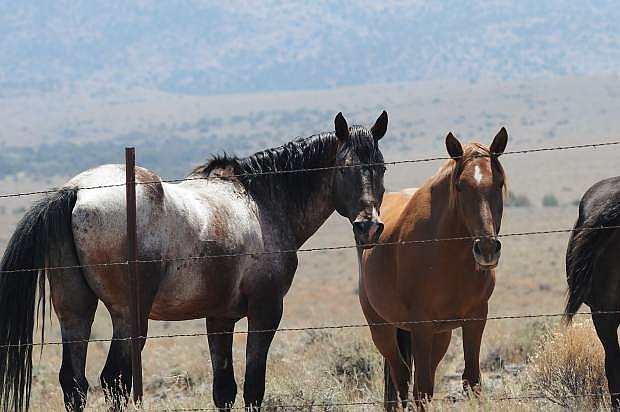In this daytime image, three horses stand in a grassy field enclosed by a rusty metal pole holding four horizontal strands of barbed wire. The field's grass is a wheat-colored brownish-green mix, extending into the distance towards large rolling hills that blend bluish and grayish hues. Dominating the foreground, from left to right, the first horse is distinct with a primarily white body marked by dark brown patches on its back and belly, complemented by black legs, mane, face, and tail. Next to it, a reddish-brown horse features a small white star on its forehead. To the extreme right, only the tail and rear end of a black horse are visible. The serene rural setting is bathed in sunlight, emphasizing the natural, pastoral beauty of the scene.